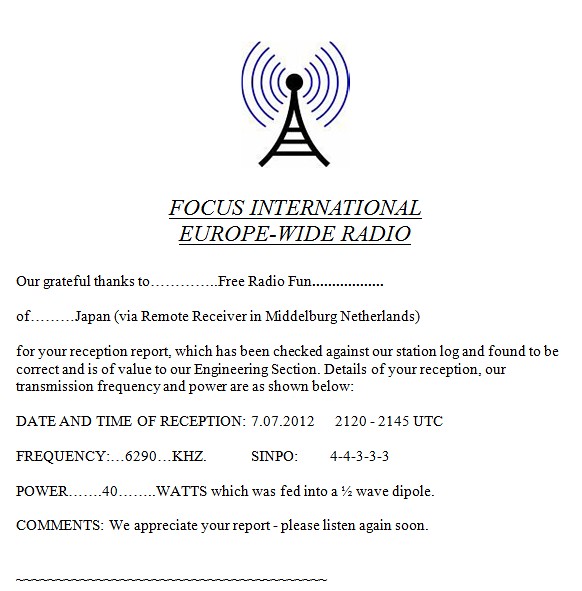The image features a black icon of a radio tower at the top, resembling an inverted triangle, emitting purple semi-circular waves. The background is white, with all the text in black. The title reads, "Focus International Europe Wide Radio." Below the title, it states: "Our grateful thanks to Free Radio Fun of Japan via remote receiver in Middelburg, Netherlands, for your reception report, which has been checked against our station log and found to be correct and is of value to our engineering section. Details of your reception, our transmission frequency, and power are as shown below." The date and time of reception are noted as 07/07/2012 at 21:20-21:45 UTC. The frequency is listed as 6,290 kHz, with a SINPO rating of 44333 and power of 40 watts, transmitted via a half-wave dipole antenna. Additional comments state: "We appreciate your report. Please listen again soon."